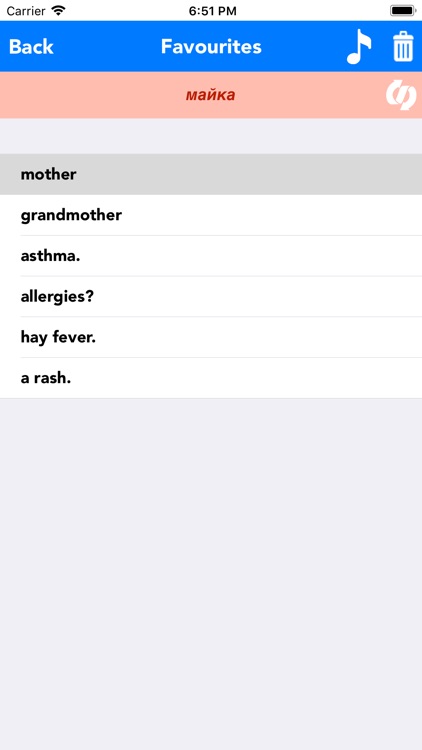Screenshot of a smartphone interface at 6:51 p.m. The phone is connected to the internet, and the battery is fully charged. At the top of the screen, there is a banner featuring a blue line on the left with "Back" written in white font, a center section with "Favourites" spelled in British English, and icons of a music note and a trash can on the right. Below this banner, the text "МАНКА" (in Cyrillic) is displayed with an icon to its right. Following this, there is a blank light gray bar, succeeded by a darker gray bar with the word "Mother" on the right side. Further down, on white bars, are the words "Grandmother," "Asthma," "Allergies?" "Hay Fever," and "Rash," each followed by a dot. At the bottom of the screen is a wide gray area that seems to be a text input field, possibly for typing information. The context of the screen suggests it could be related to health or personal notes, though the exact purpose is unclear.